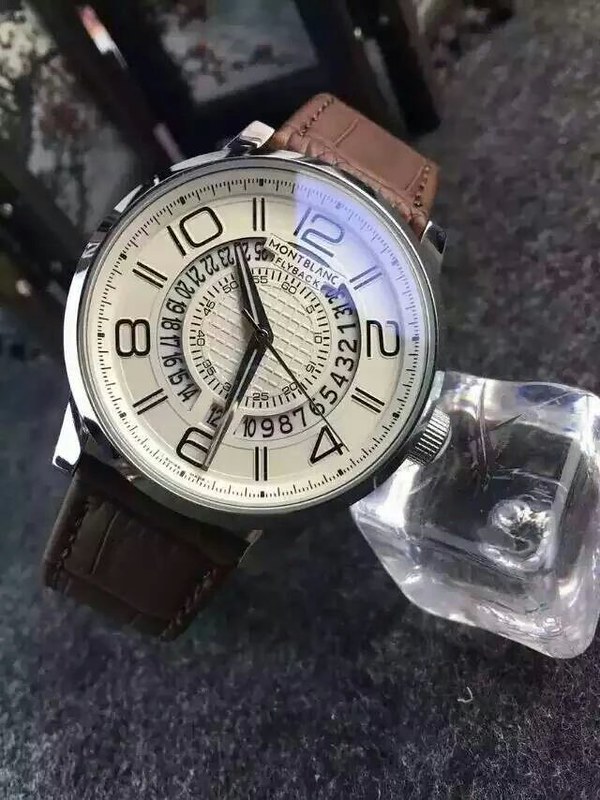This close-up, detailed photograph features a sophisticated men's Montblanc watch, elegantly positioned against an ice cube on a textured, gray, fibrous surface. The timepiece boasts a large silver-rimmed face with a beige background, highlighted by bold black numerals representing the even hours: 12, 2, 4, 6, 8, and 10. The odd hours are indicated by subtle hash marks. Minute and second markings adorn the interior section of the watch face near the point where the hands are anchored. The watch currently shows the time as 10:30, with the second hand precisely on the 20-second mark. Completing its refined appearance, the watch features a rich brown leather band and has additional millisecond hash marks encircling its perimeter, emphasizing precision and attention to detail.